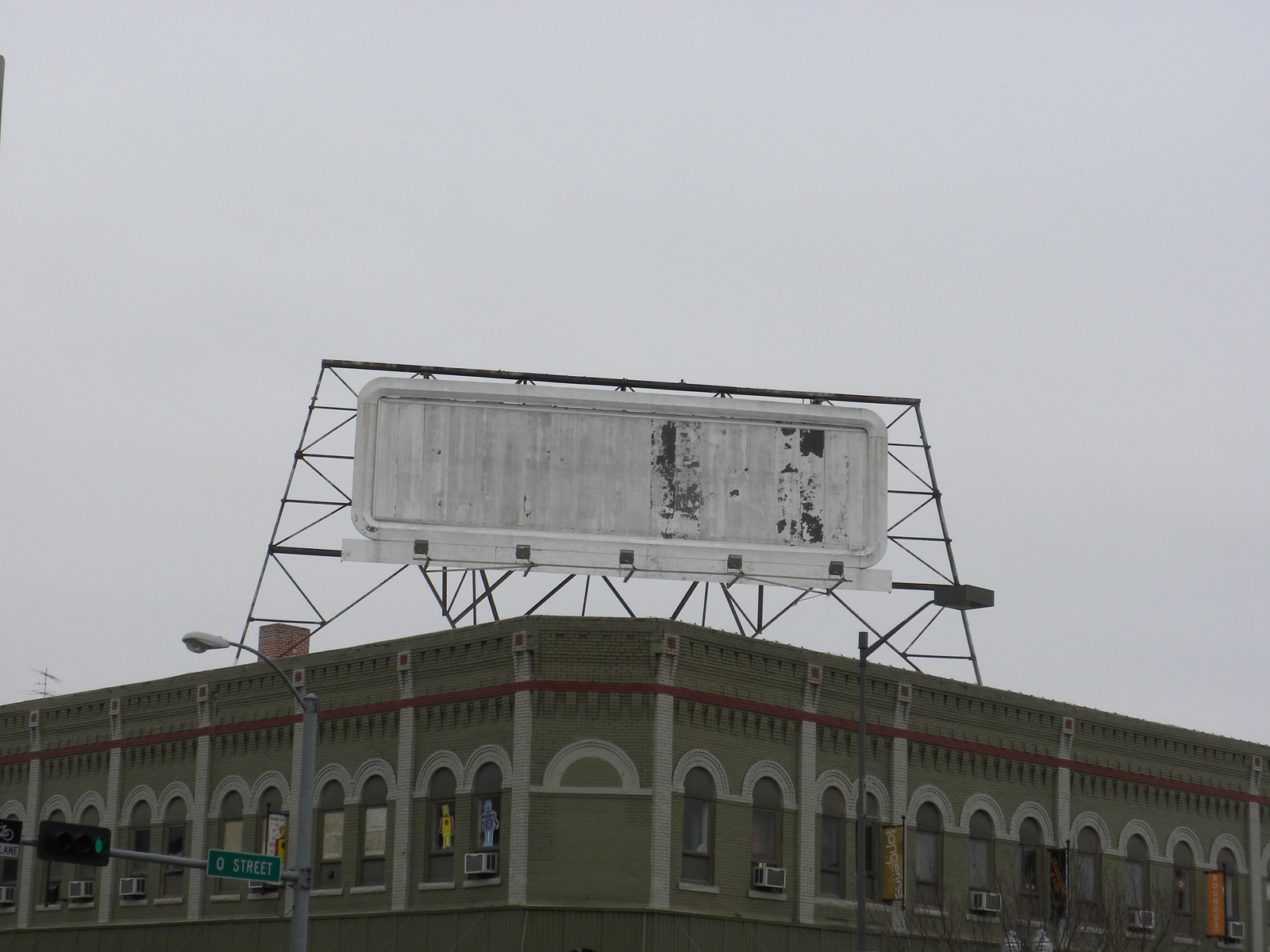The photograph depicts a green concrete or stone building situated on a corner, where the two sides meet. The building features arched windows reminiscent of church architecture, adorned with white designs above them. A notable red stripe accents the very top of the structure. At the building's apex, there is an empty white rectangular billboard mounted on a black triangular scaffold, indicating the remnants of a previous advertisement. The scene is captured on an overcast day, with a gray, almost blue, sky. In the bottom left corner of the image, a green street sign and traffic light are visible, indicating Zero Street with the light currently green. Air conditioners are seen protruding from some of the windows, enhancing the urban aesthetic. The overall color palette of the photograph includes greens, grays, blacks, and whites.